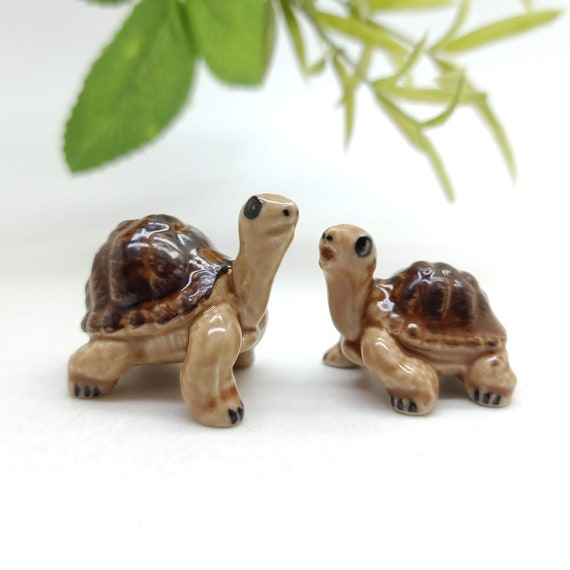This is a close-up photograph of two small decorative ceramic turtles. Both figurines feature dark brown, high-domed shells that appear glossy, and they are positioned on a featureless, white surface. The turtles have lighter beige-brown bodies, with tiny black claws on their feet, and subtly detailed black eyes. The turtle on the left has its neck outstretched slightly more and mouth closed, giving it a composed expression, while the one on the right has a shorter neck and a slightly open mouth, which makes it look surprised. Both turtles are facing each other in the frame. In the blurred background, a variety of plant leaves can be seen, some quite broad and others narrow, adding a touch of natural ambiance to the image. The overall setting suggests an ornamental or decorative context, likely suitable for an online catalog or sales listing.